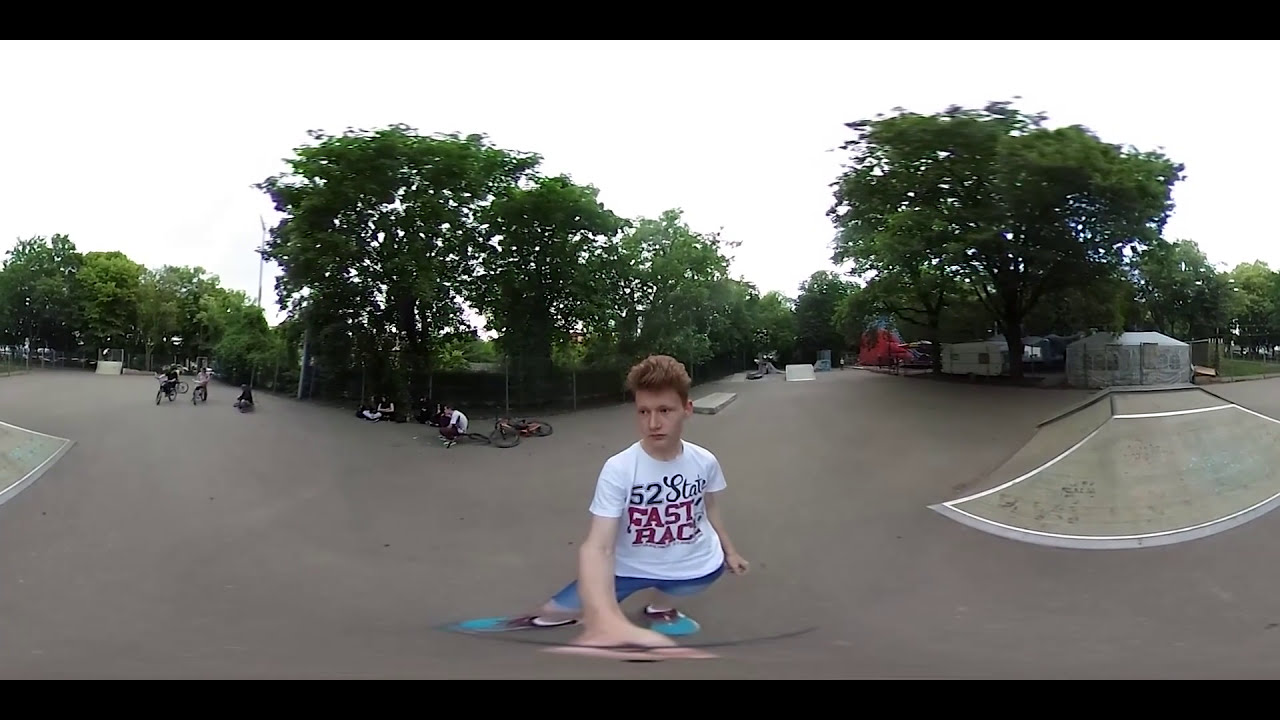The photograph captures a young man at the center of a bustling outdoor BMX or skate park. He stands poised on a light gray asphalt surface, ready to create a panoramic selfie. He is outfitted in brown shoes with white ankle socks, short blue denim pants, and a white short-sleeved crewneck graphic t-shirt reading "52 stars, fast, race." With short, fluffy light brown hair, the young man gazes to his right, adding a candid touch to the scene. The park around him is lively—on the left, several people lounge or sit near an array of bicycles scattered on the ground, while others ride in the background. The sky, a light gray, frames the rich, dark green trees behind him, providing a picturesque backdrop. To his right, a small ramp punctuates the setting, enhancing the park's dynamic atmosphere. The photograph's lens creates a unique, oblong effect, emphasizing the proximity of objects and the panoramic intent of the young photographer.